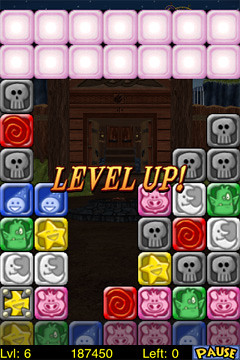This screenshot captures a vibrant moment from a block-busting game app, where players combine identical shapes to make them disappear. The rectangular image is divided into sections, with the topmost portion featuring two rows of squares, 14 in total – 7 on the top row and 7 on the bottom row. Each square contains a unique shape, including a gray skull, a red spiral, a blue square with smiley faces, a pink pig, and a moon, adding a playful diversity to the game's design.

Dominating the center of the screen, "LEVEL UP" is prominently displayed in large, bold yellow letters, celebrating the player's progress. At the bottom of the screenshot, "Level 6" is shown in the bottom left corner, indicating the current stage. Centrally placed just above the bottom edge, "Left: 0" indicates that there are no shapes left to pop for that level. Finally, "Pause" is written in a curved font positioned at the bottom right, offering players a moment to take a break from the action.